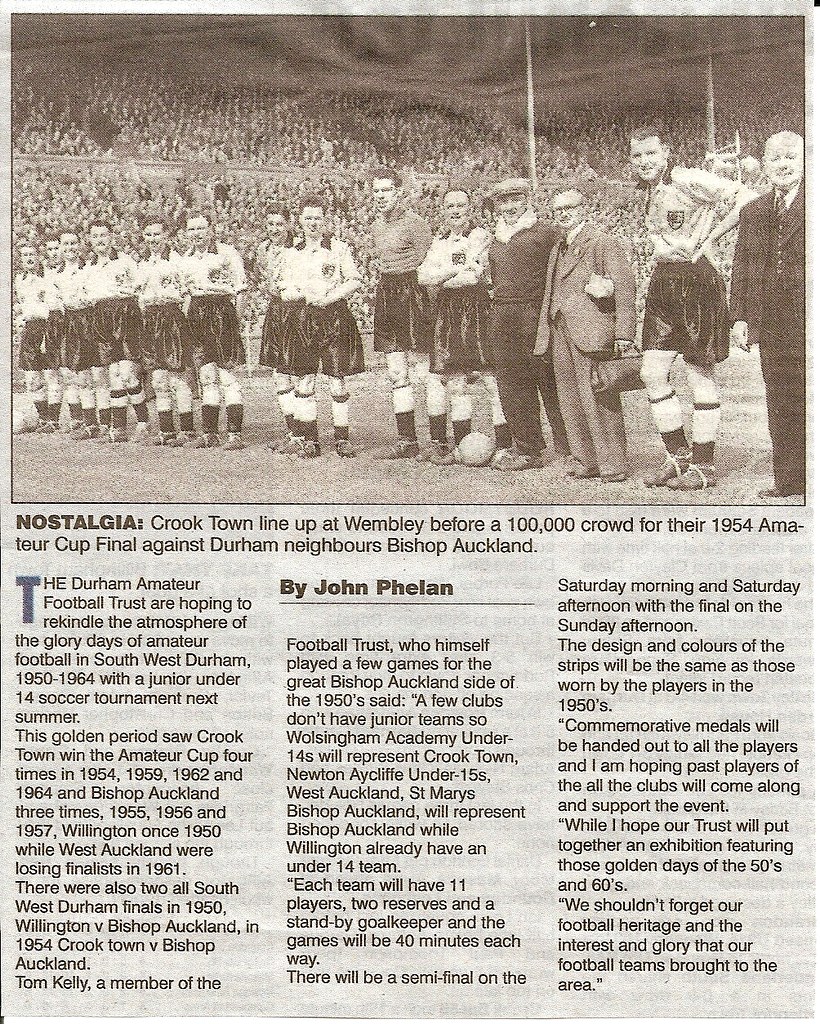The photo depicts an old English football (soccer) team from a 1954 newspaper article. The black-and-white image shows the Crooktown team lined up in a row at Wembley Stadium, dressed in white shirts with dark collars and dark shorts, with management in suits standing beside them. They are preparing for the 1954 Amateur Cup Final against Durham neighbors Bishop Auckland, before a massive crowd of 100,000 spectators. The background features a filled stadium. Below the image is a three-column article by John Palin detailing the tournament events, with the byline prominently displayed in bold black text.